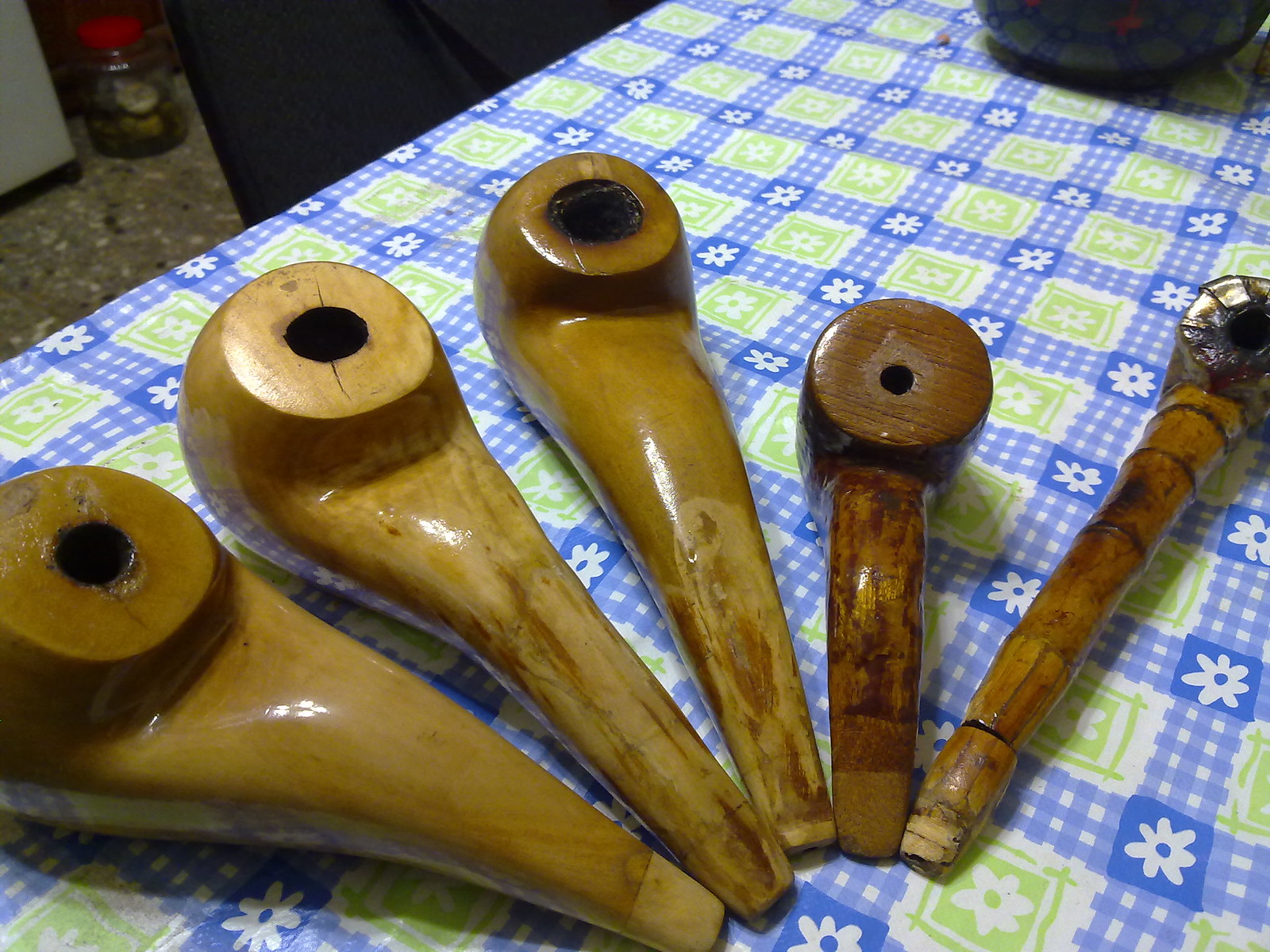The image features five rustic, handcrafted wooden pipes, displayed on a blue, white, and green plaid tablecloth adorned with white floral patterns. The pipes, likely designed for smoking tobacco or perhaps marijuana, are arranged in a radial pattern, with their mouthpieces touching near the center-right of the image. Each pipe is unique in shape and size, yet they all share some common characteristics: a wide cylindrical bowl, char marks indicating use, and variations in wood color and finish.

From left to right, the first pipe has a broad, round shape that tapers to a point, with a darker wood circular hole at the top. The next two pipes share a similar shape but are more distressed, with the third one being slightly thinner. The fourth pipe stands out with its darker brown wood, shorter handle, and more hammer-like shape. The final pipe, markedly different from the rest, is long and thin, featuring a medium brown wood with a dark brown circular end. In the background, a jam jar with a red lid can be seen, adding a touch of everyday life to the otherwise esoteric collection.